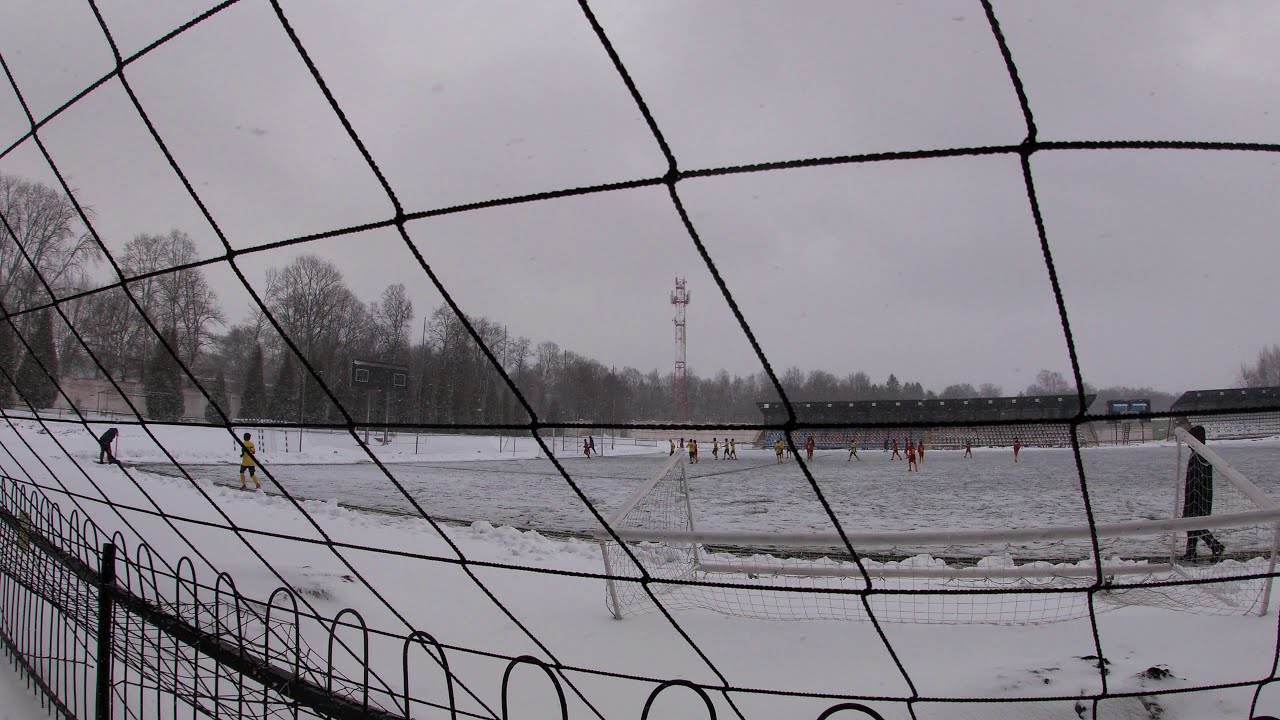The photo captures a wintry scene on a gloomy day, taken from behind some black netting and a low black fence that curves towards a circular shape in the lower left corner of the image. The foreground and surrounding area are blanketed with snow, indicating a cold, snowy environment. The scene appears to be of an ice skating rink, possibly set up for hockey, with several tiny figures in the distance wearing what look like yellow and red jerseys, engaged in some sort of sport.

Beyond the rink, there's a snow-covered walking path and another snow-covered area to the left. In the background, a tree line of barren deciduous trees, along with a few pine trees, stretches across the horizon. Amidst the trees, a tall tower, possibly a 5G tower, stands prominently against the dark gray sky, which hints at ongoing snowfall.

On the opposite side of the rink, there are bleachers for spectators, and between two sets of bleachers, an unlit scoreboard can be seen. The overall atmosphere is that of a quiet, snow-covered sports arena, surrounded by winter's stillness and the distant trees marking the boundary of the scene.